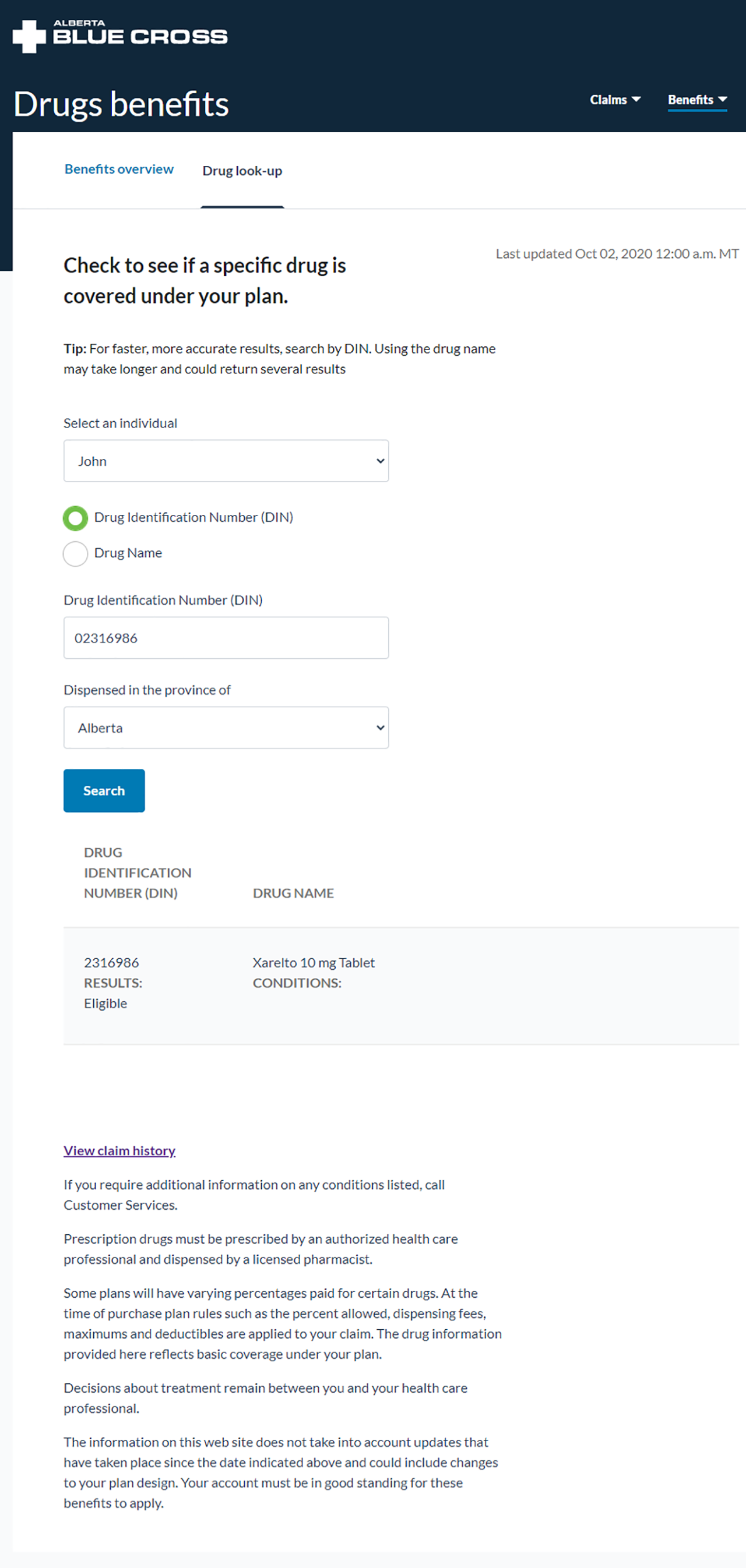The image displays a webpage for Alberta Blue Cross, a healthcare provider in Canada, focusing specifically on drug benefits. 

At the top of the page is the header that reads "Alberta Blue Cross," with a small white cross icon to the left. The word "Alberta" is smaller in size compared to "Blue Cross." Directly beneath the header is the title "Drug Benefits."

To the right, there is a navigation element with a drop-down box labeled "Claims," and the "Benefits" option is currently selected and highlighted in blue. Below the "Drug Benefits" header, on the left side, there is a section for "Benefits Overview" and "Drug Lookup." The "Drug Lookup" tab is currently active and underlined.

The description under "Drug Lookup" reads: "Check to see if the specified drug is covered under your plan." On the right, there is a note stating the last update of the page: "Updated on October 2nd, 2020 at 12 a.m."

Moving further down, there are tips in smaller text advising users to search using the Drug Identification Number (DIN) for faster and more accurate results, as using the drug name might take longer.

The section proceeds to show options for selecting an individual (currently showing 'John') and whether to search by drug ID number or drug name. The search by drug ID number is selected with a green button. Below this, there is a field for entering the DIN, followed by an option to select the province, defaulted to Alberta, and a blue search button.

The results section displays the Drug Identification Number along with additional information about the drug, such as its dosage in milligrams. There is also an option to view the claim history. At the bottom, there is a standard disclaimer statement.